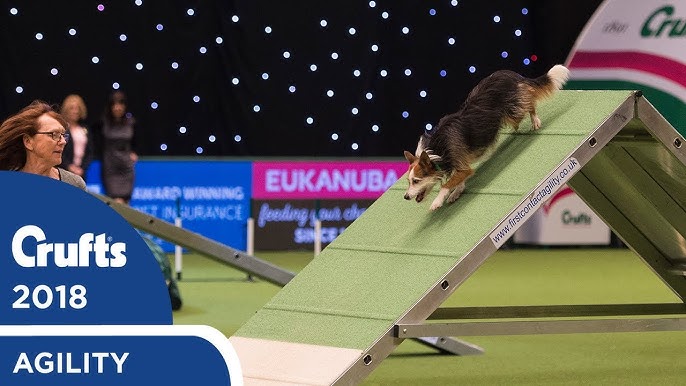This image showcases a thrilling moment at the Crufts 2018 dog show, specifically within the agility section. A small, tri-colored Border Collie, displaying hues of white, tan, and black, is captured mid-action as it navigates down a green AstroTurf ramp with silver sides. The ramp features some advertising, indicative of sponsorship. To the left of the frame stands the dog's trainer, a woman with glasses and reddish hair, intently focused on guiding her canine companion. The backdrop reveals a flurry of activity, with studded black and white displays adorned with various advertisements including those for Eukanuba and an insurance company, some partially obscured. Additionally, the event signage is prominent, with "Crufts 2018" and "Agility" highlighted in white font on a navy blue background. In the distance, two judges observe the performance, ensuring fair play in this high-stakes competition. The atmospheric scene is accentuated by the presence of blurred sponsor signs and spotted lights, adding to the ambiance of this prestigious dog show.